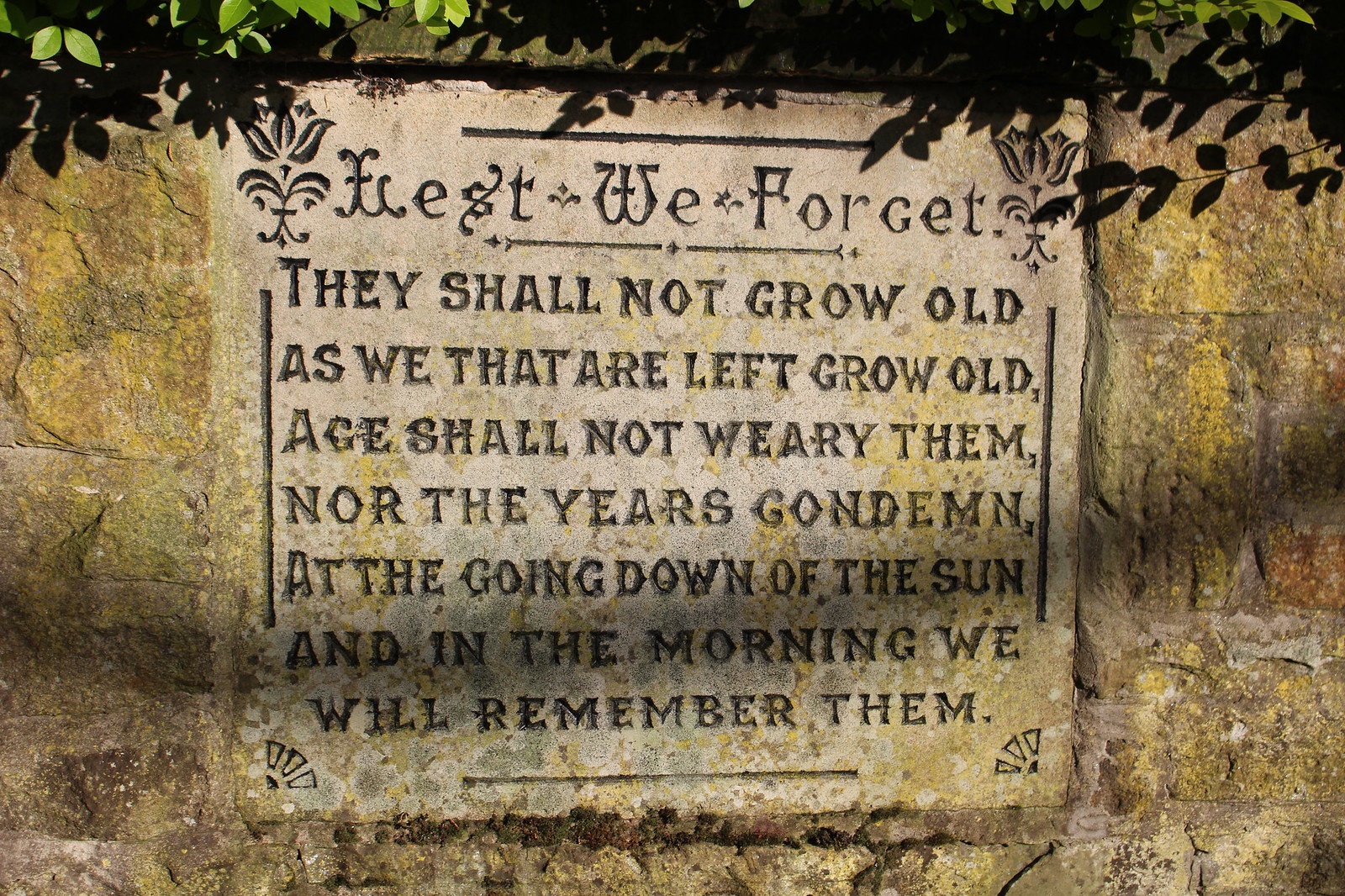The image depicts a memorial with a prominently placed gravestone in the center of the frame, standing against a weathered stone background. Surrounding this central stone, which features an intricate carving, are various bushes and leaves that adorn the top portion of the photo. The smooth surface of the gravestone is engraved with a poignant inscription in elegant, capitalized font: "Lest we forget. They shall not grow old, as we that are left grow old; age shall not weary them, nor the years condemn. At the going down of the sun and in the morning, we will remember them." This quote is meticulously carved into the stone, with letters appearing in brown or dark gray. The gravestone is slightly accented with patches of yellow moss, indicating its age. The scene appears to be outdoors, possibly by the side of a building, captured in the clear light of midday. The visible colors in the image include various shades of green, yellow, brown, gray, black, and tan.